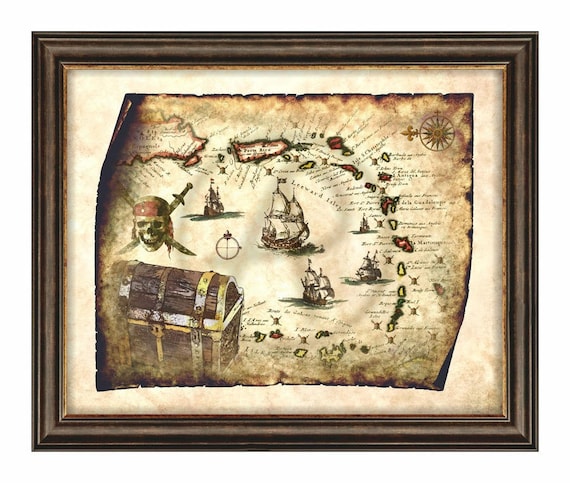This picture, framed in a dark brown wooden frame, showcases a meticulously designed, aged-looking pirate treasure map. The main image, sitting on a cream-colored matte background, appears to be a computer-generated replication made to look historic and tattered, complete with blackened, torn edges and a generally brown, rusty hue. The map itself features a rich array of pirate-themed elements: a large treasure chest in the bottom left, an ominous pirate skull with a red bandana and two crossed daggers above it, several grand sailing ships in the center, and a compass in the top right. Surrounding the ships, approximately ten islands are depicted in a circle, with detailed, albeit small and unreadable, text describing the geography of these islands. This intricately framed artwork captures the essence of pirate lore and treasure hunts, evoking an adventurous, ancient maritime atmosphere.